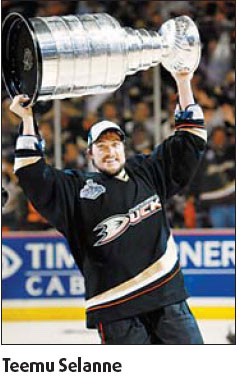This vertically oriented photograph showcases a jubilant hockey player named Teemu Selanne, as indicated by the name inscribed at the bottom of the image. Selanne is exuberantly holding an enormous silver trophy, likely the Stanley Cup, aloft with both hands, showcasing the moment of triumph. He is dressed in a black hockey jersey emblazoned with the word "Ducks" in bold white lettering, accompanied by a significant yellow-gold logo. His attire includes a white cap and what appears to be black hockey pants or sweatpants. Teemu's appearance features brown hair and a medium-sized brown beard, and he is captured smiling broadly in mid-celebration. The photo is cropped at mid-thigh, focusing on the upper two-thirds of his body. The background reveals the atmosphere of an ice rink, complete with a blurred crowd of cheering fans, advertisements, and a little blue banner along the rink's side, encapsulating the essence of a victorious moment in the sport's arena.